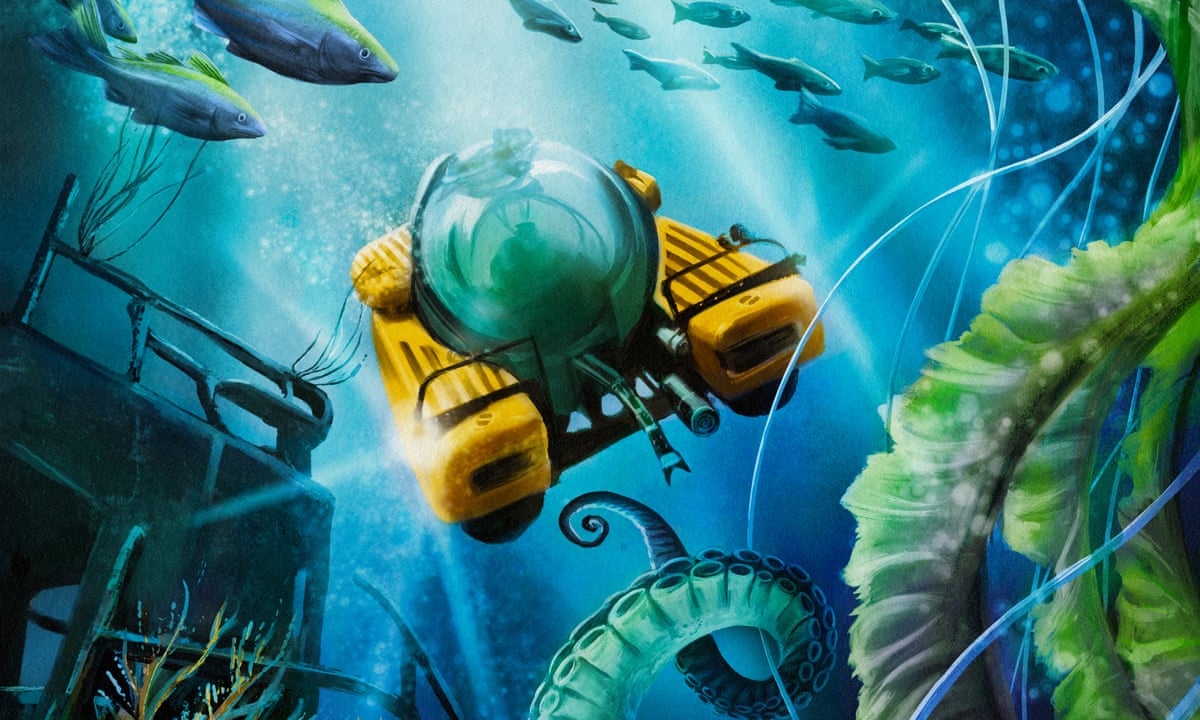The image depicts a richly detailed underwater scene illustrated in an animation or book-style drawing. Central to the image is a large, glass orb submarine, equipped with prominent yellow contraptions on its sides and illuminated by lights, enabling an undersea explorer to journey into the depths safely. Surrounding the submarine, intricate elements of aquatic life are vividly portrayed: a sinuous octopus tentacle curls upwards in the middle frame, while vibrant green seaweed tendrils sway gently to the right, releasing air bubbles that rise towards the surface. At the top of the image, against a backdrop of beautiful blue water, about nine to ten schools of fish swim to the right, illuminated by rays of light streaming down from above. In the lower left, an abandoned piece of dilapidated metal, possibly part of a sunken truck or similar wreckage, rests eerily on the ocean floor, adding to the sense of underwater mystery and exploration.